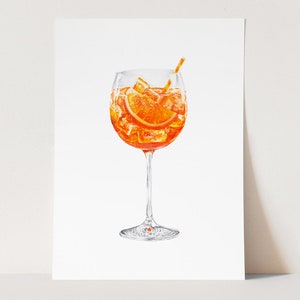This image depicts a detailed artwork, possibly a painting or a computer-generated graphic, propped up against a neutral white wall. The artwork is on a large piece of white paper or canvas, creating a mostly white background that casts subtle shadows down and to the right. Central to the composition is a tall, crystal-clear wine or sangria glass with a shiny appearance, filled three-quarters up with vibrant orange liquid, likely a type of cocktail. Several ice cubes are visible, some near the bottom of the glass and others floating towards the back, providing a sense of depth. In the middle of the drink, positioned at a slight angle, there is a fresh orange slice, adding a splash of color and a hint of flavor to the depiction. Emerging from the top right of the glass is an orange straw with white stripes, contributing a playful touch to the scene. At the very bottom of the glass, right at the base, a small red dot is noticeable, adding an intriguing detail to the artwork.